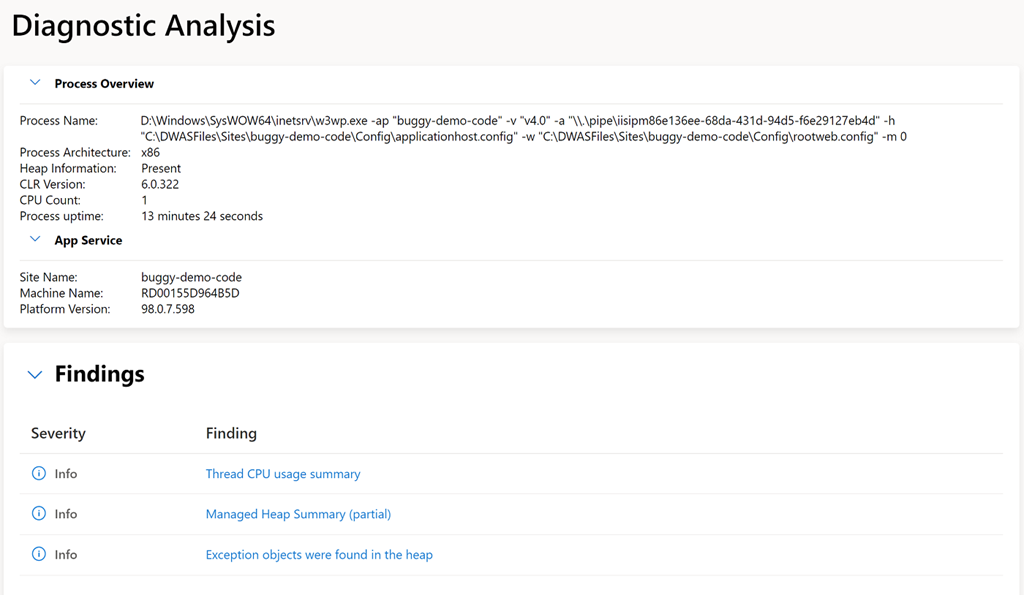**Caption:**

The image displays a diagnostic analysis report on a white background. At the top left, the title "Diagnostic Analysis" is prominently displayed. Directly below is the header "Process Overview," accompanied by a blue down arrow to its left. Following this is a section labeled "Process Name," specifying the computer file path for the process. Important details listed under this section include:

- Process Architecture: x86
- CLR Version: 6.0.322
- CPU Count: 1
- Process Uptime: 13 minutes 24 seconds

Further down, another header labeled "App Service" with a blue down arrow beside it introduces additional information including:

- Site Name: Buggy-Demo-Code
- Machine Name: RD00155D964BSD
- Platform Version: 98.0.7.598

A larger section titled "Findings," also marked with a blue down arrow on the left, is present towards the bottom of the image. Under the "Severity" label, all items are marked as "Info" with a blue information icon preceding each. Detailed findings listed include:

- Thread CPU Usage Summary
- Managed Heap Summary (Partial)
- Exception Objects were found in the heap

These findings are highlighted in blue, drawing attention to the diagnostic insights provided.